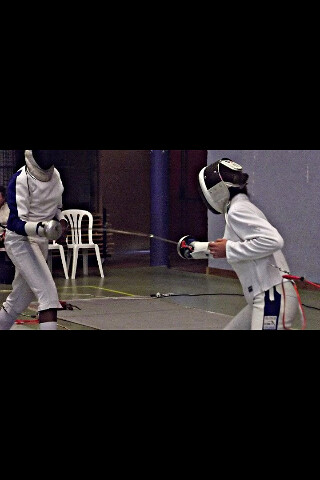The image is a small photograph, about two inches by two inches, showing two people engaged in a fencing duel inside a gymnasium. The fencers are dressed in standard white fencing gear that includes pants and tops, with helmets covering their faces. One fencer, potentially an African American individual, has a black stripe down the side of their outfit, while the other, possibly of Asian or Caucasian descent, features a blue stripe down their arm. Both are poised with their right hands pointing their swords at each other and their left hands curled in a V-shape. The gymnasium background includes a blue foam-covered pole, several white plastic chairs, and a cord strung across the space. The flooring appears to be the rubber-type often found in school gymnasiums. This setup suggests they might be practicing or taking lessons. The image itself is a screenshot from a video playing on a phone held in portrait orientation, making the visual details concise but clear.